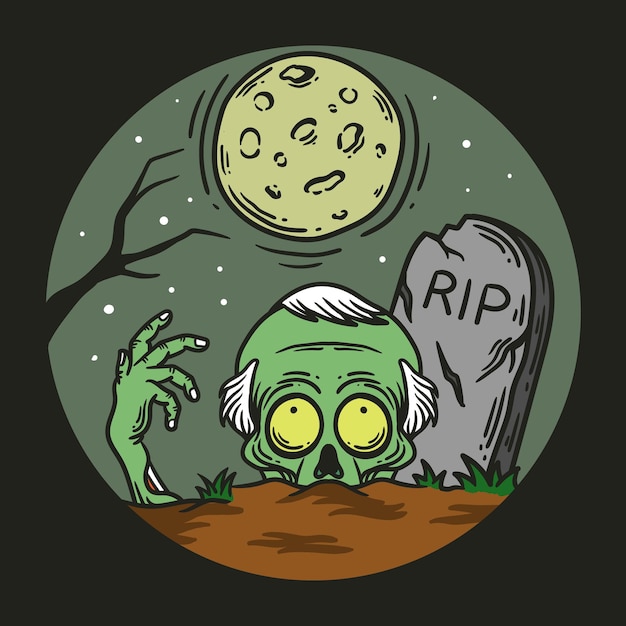This is a clip art-styled digital artwork of a green zombie emerging from the ground, set against a black square background. The central circular artwork features a night scene with an olive green sky and a full moon marked with pockmarks, giving it a cheese-like appearance, alongside several white dots depicting stars. A skeletal black tree branch reaches in from the left side. The foreground shows bright brown cartoonish soil with three clumps of green grass. The zombie's head, characterized by large yellow eyes and three tufts of white hair, pokes out from the soil up to its nose cavity. To the left of the zombie head, a clawed, partially decomposed hand rises from the ground, revealing bones and tendons. Behind the zombie, a cracked gravestone reads "R.I.P." This detailed, non-photorealistic artwork encapsulates a spooky yet whimsical scene.